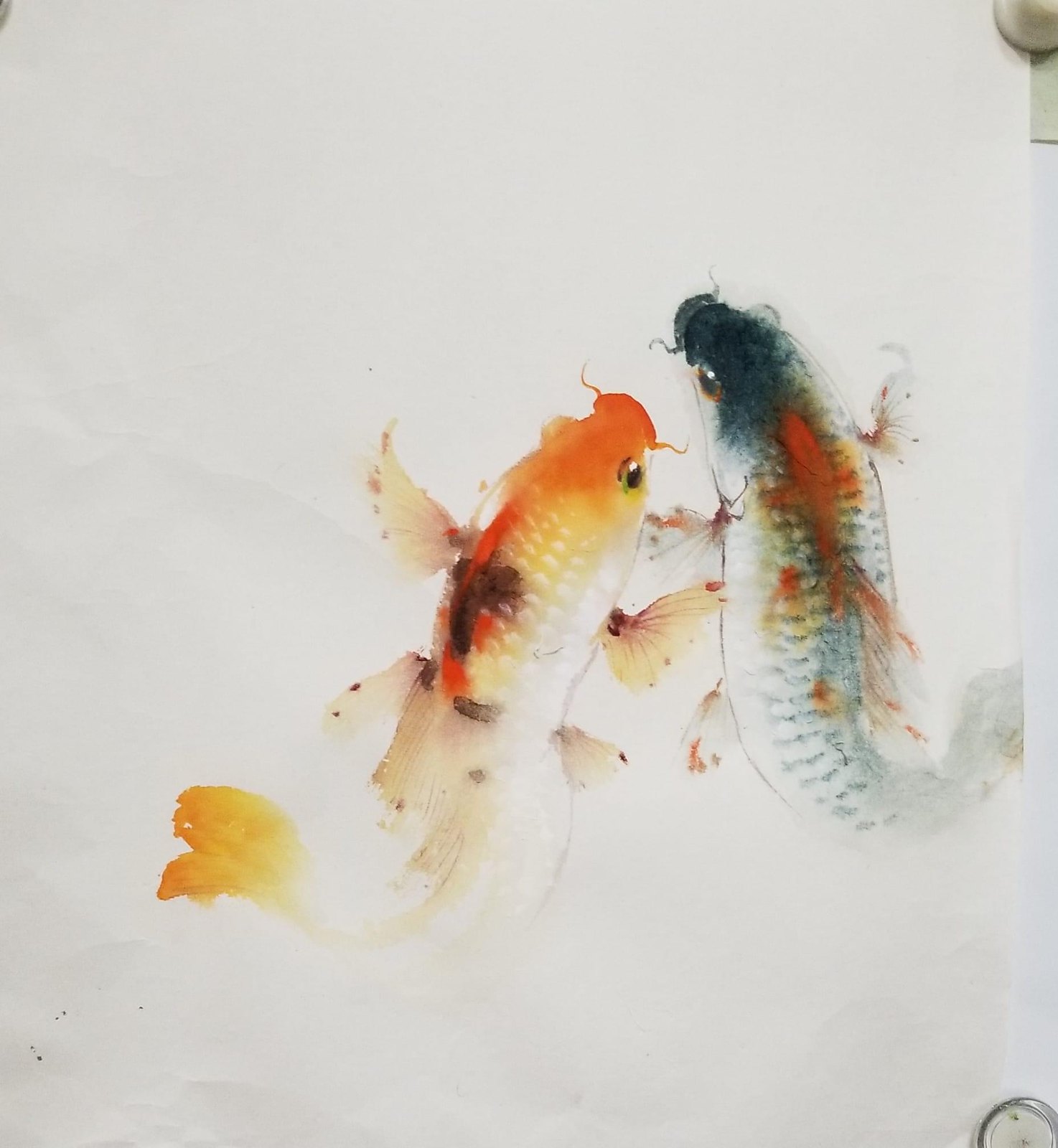This image showcases a beautifully detailed watercolor painting of two koi fish, set against a light grayish-white background. The artist has captured the fish from a top-down perspective, highlighting their distinct features and intricate details. Both fish are positioned centrally, with one slightly towards the right. 

The first koi, occupying the center with its tail extending to the left, has a primary white body adorned with splotches of dark orange, light orange, and yellow, and a distinctive brown spot on its back. The fish’s fins are elegantly outstretched as it swims with a gentle curve, and its tail gradually transitions from orange to yellow and then white.

On the right side, the second koi combines an array of colors, beginning with a predominantly white body that transitions into light blue with dark blue accents. This fish features a striking black patch on its head, while its fins exhibit gold hues. The body displays a mix of light gray and white tones along with an orange stripe, adding to its dynamic appearance. Like its counterpart, this fish appears to be swimming gracefully, with its tail extending towards the right of the painting.

Subtle reflections of light on the fish’s bulging eyes and the delicate whisker-like tendrils near their mouths add to the realism of this aquatic scene. The slight wrinkles and the appearance of the paper suggest it may be held in place on a board or refrigerator by magnets, adding an authentic, personal touch to the artwork.